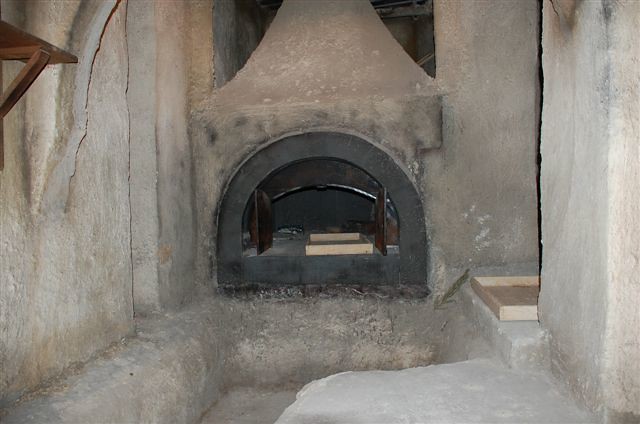The image showcases an outdoor, semi-circular shaped, pizza oven-like fireplace nestled within a partially visible concrete and stone structure. The oven features two small doors and is framed in a burnt-out black color, with darker brown tones. The interior of the fireplace is blackened, likely from soot and use, and sits empty except for a light wooden tray placed inside. The stone facing around the front of the fireplace is gray with accents of light brown, showing signs of weathering and soot markings, along with some red accents at the top. This fireplace structure, which includes a black metal frame around the top and bottom, is part of a stucco room with built-in seating around it. The stone chimney above the fireplace extends upwards, and there is a wooden shelf on the left side near the top, supported with a wooden bracket. The front area of the fireplace is flanked by stone walls and pillars, with stone flooring extending around it.